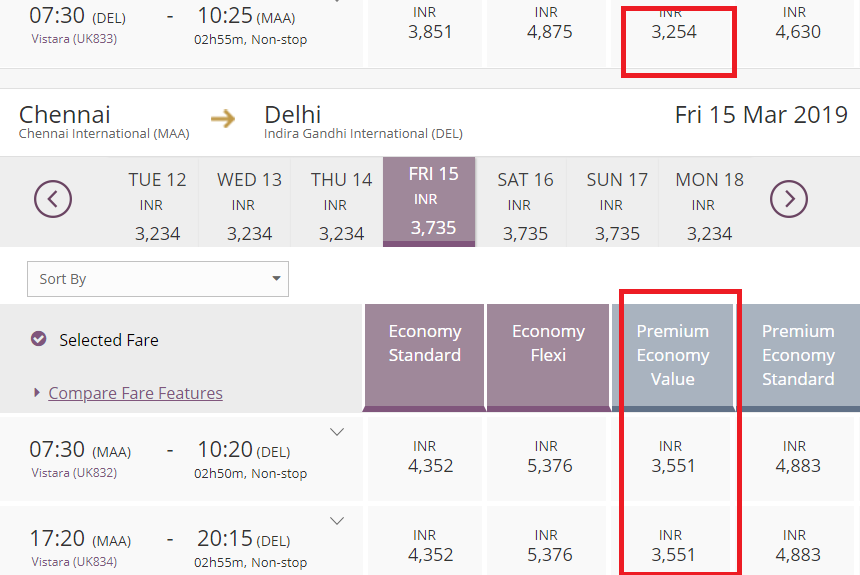This image displays detailed flight plans for two routes involving Indira Gandhi International Airport (DEL) in Delhi and Chennai International Airport (MAA). 

At the top of the image, a flight is scheduled to depart from Delhi (DEL) at 07:30 AM via Vistara and is expected to arrive in Chennai (MAA) at 10:25 AM, covering a non-stop duration of 2 hours and 55 minutes. The prices for this flight are listed in Indian Rupees (INR), with the following fare options: ₹3851, ₹4875, ₹3254 (highlighted in red), and ₹4630. 

The second flight route is from Chennai International Airport (MAA) to Delhi Indira Gandhi International (DEL), dated Friday, March 15th, 2019. The sorted fare screen shows selected prices for this flight as well, facilitating a comprehensive comparison. 

The fare comparison includes various categories such as Economy, Economy Flex, Premium Value, Economy Value, and Premium Economy Standard, with their respective costs and features displayed. Among the options provided, the Premium Economy Value is highlighted as the best choice in terms of cost-effectiveness for both routes.